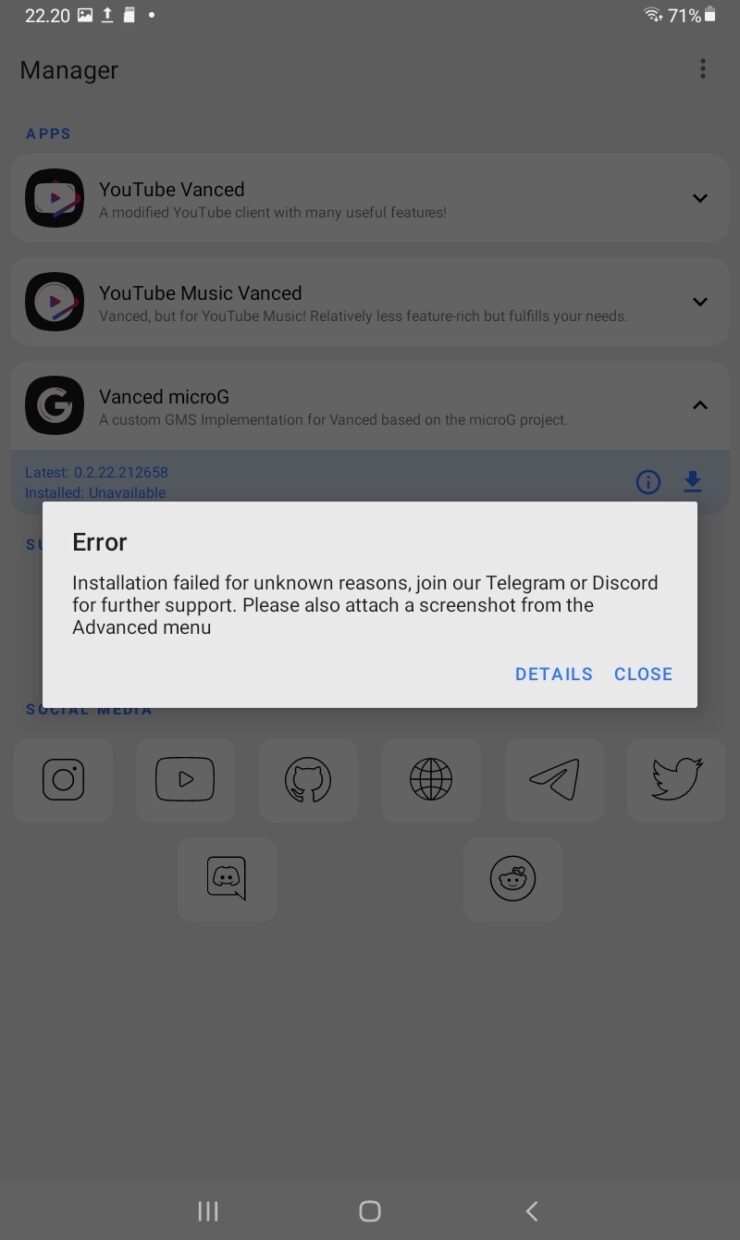**Screenshot of Android Device Displaying App Manager with Installation Error**

This screenshot, captured from an Android device, displays the App Manager screen with specific details. At the top-left corner, the time is shown as 22:20, while the top-right corner exhibits various status icons, including a battery indicator at 71%. The title "Managers" is prominently displayed at the top. Directly beneath this title, the "Apps" section lists three applications: YouTube Vanced, YouTube Music Vanced, and Vanced MicroG.

Central to the screen is an error message stating, "Installation failed for unknown reasons. Join our Telegram or Discord for further support. Please also attach a screenshot from the advanced menu." This message suggests a failure during the installation process of one of the listed apps.

At the bottom of the screen, multiple social media icons are visible, providing links to Instagram, YouTube, GitHub, the web, Telegram, Twitter, Discord, and Reddit for additional support and community interaction.

The screenshot also shows the typical Android navigation buttons at the very bottom of the device screen. Overall, the image indicates that the user is facing difficulties installing an app and is directed to seek assistance via social media platforms.